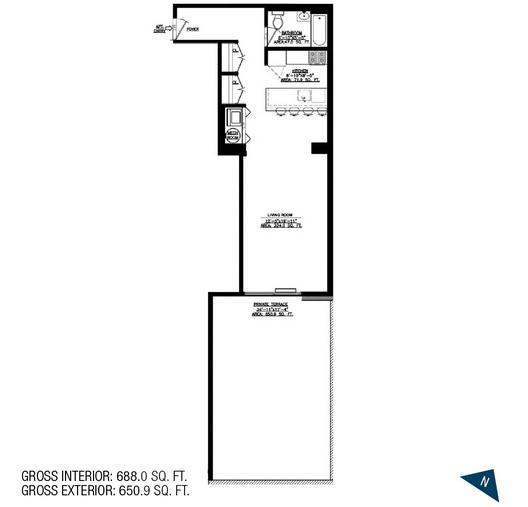This is a detailed floor plan of a long, narrow building with a gross interior area of 688.0 square feet (SQ. FT.) and a gross exterior area of 650.9 square feet. The schematic is presented on a white background, which is predominant throughout the image. 

In the bottom right corner of the plan, there is a blue triangle featuring a white letter 'N', indicating north and pointing towards the northeast direction on a traditional map. On the bottom left, there are annotations detailing the interior and exterior square footage.

The building comprises a narrow layout with a restroom located at the topmost portion, featuring a toilet, sink, and bathtub along with an unidentified fixture. Adjacent to the bathroom is a kitchen area, sharing a common wall. The kitchen appears to be a galley style, equipped with cabinets, a stove top, a sink, and a countertop that doubles as a bar seating area.

Multiple doors are visible, though the exact labeling and additional details are challenging to decipher due to small text. The floor plan transitions from a long, narrow rectangle at the top to a broader, shorter rectangle at the bottom, suggesting either a continuation of the main floor or a different level entirely. The overall design hints at either a compact house or a small business space, though the exact function remains unclear based on the current information.